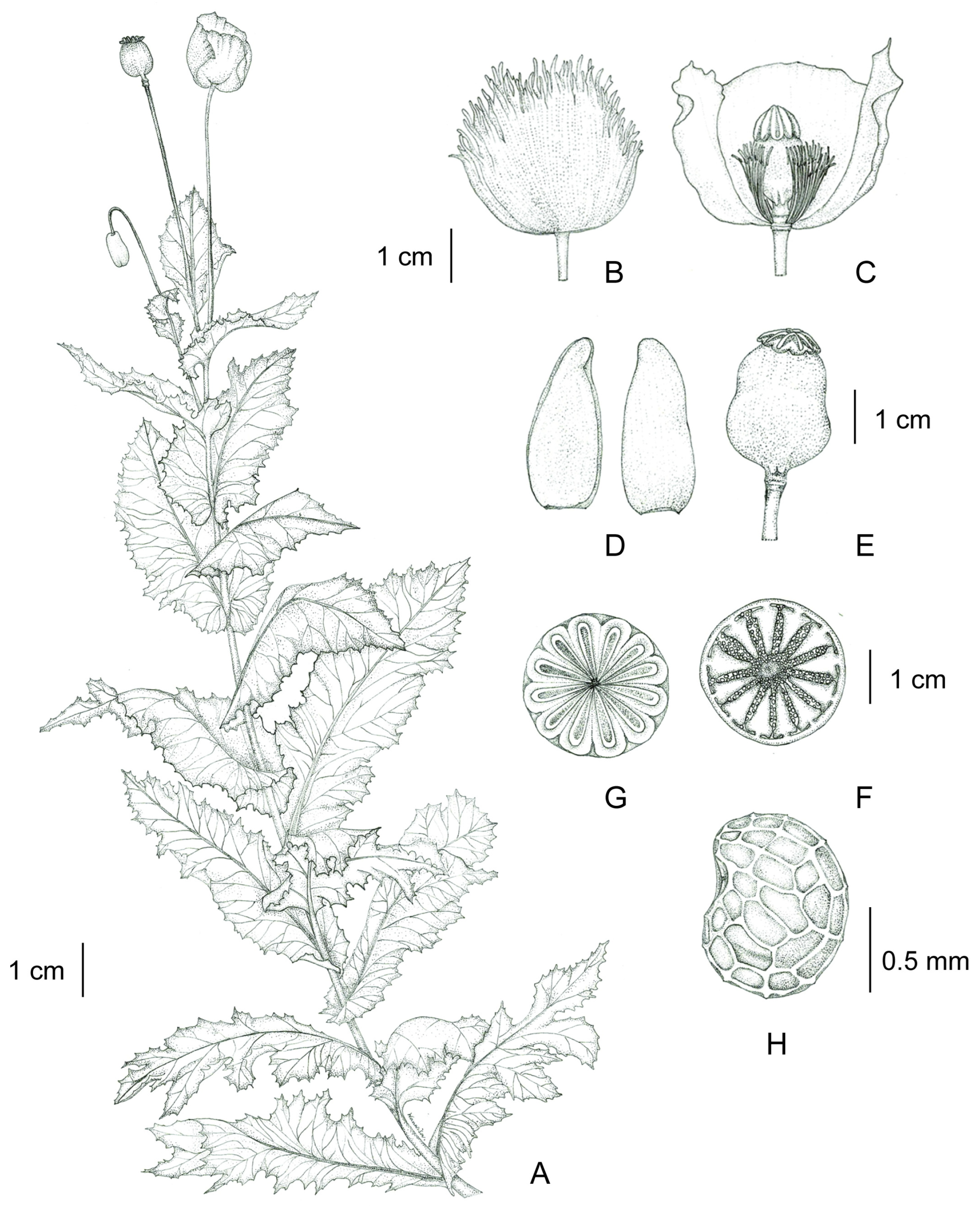This is a detailed black and white illustration of a plant, meticulously drawn in pencil, set against a plain white background without visible borders. The entire plant, labeled as 'A', stands about six inches high and four inches wide and features a long, slender stem with numerous elongated, spiked leaves that taper as they ascend. At the top, there are three buds: one fully closed, one curved over, and the third partially opened. To the lower left of illustration 'A', there is a scale marker reading one centimeter.

To the right, a series of detailed drawings span from top to bottom, illustrating various parts and stages of the plant, labeled B through H. Figure 'B' depicts the external view of a bud, while 'C' shows an internal view, revealing the intricate structure inside the bud. Both images are accompanied by a one-centimeter scale for reference.

Further down, 'D' shows two bean-shaped petals, and 'E' illustrates these petals combined on a stem. Both images include a one-centimeter marker.

At the bottom, figures 'F' and 'G' present two circles with different internal structures; 'F' resembles a wagon wheel with spokes, and 'G' looks like elongated petals, akin to the segments inside an orange, both also marked with a centimeter scale.

Finally, 'H', at the very bottom, displays another bean shape with small oblong shapes inside it, and is marked with a 0.5 millimeter scale, highlighting the minute details of the plant's structure. This comprehensive diagram captures the full morphology of the plant, from the entire structure to the intricate details of its parts.